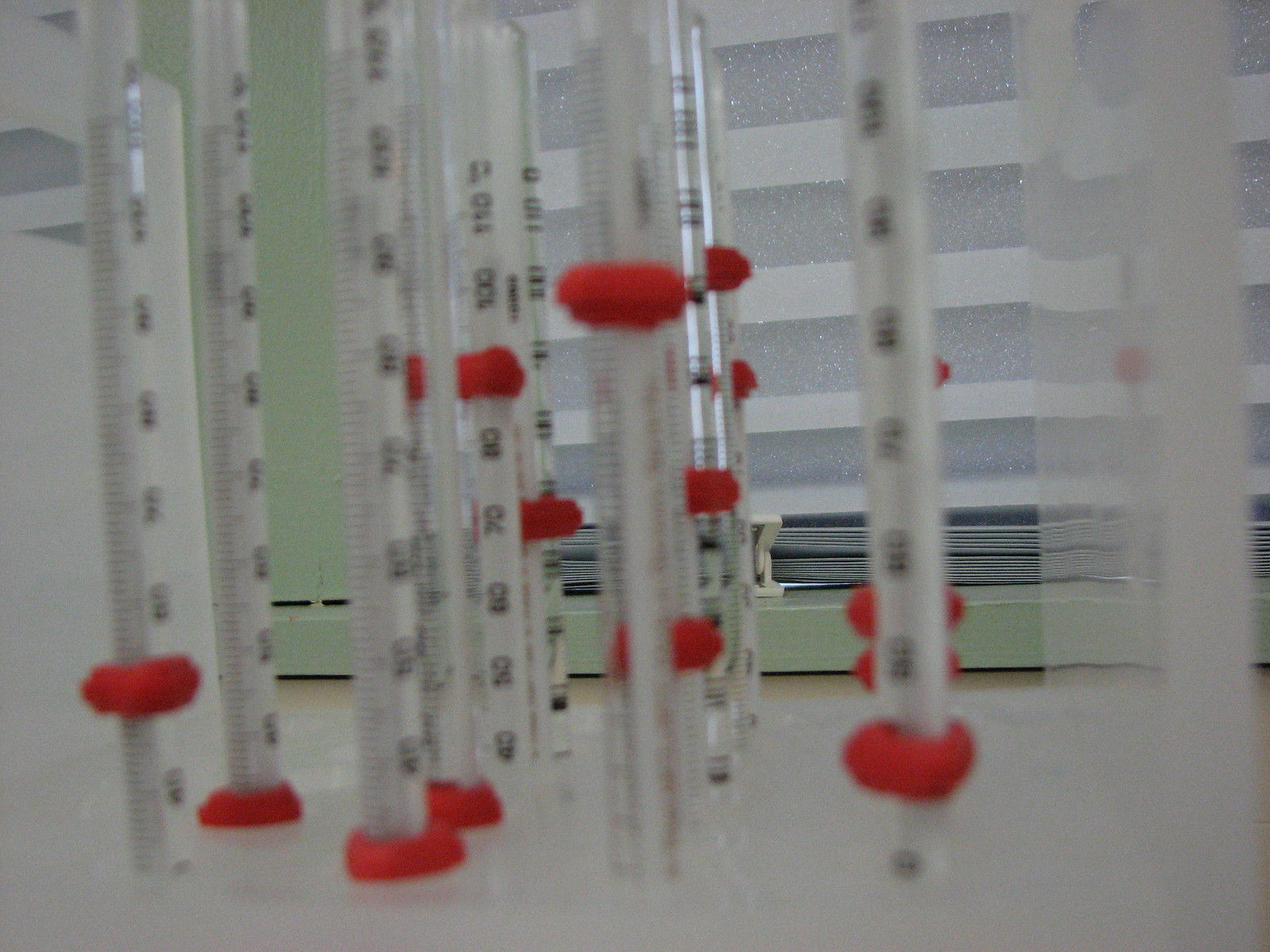The image is slightly blurry, depicting a row of nine or ten upright thermometers with red bases and clear tubes. Each thermometer is marked with numbered intervals: 40, 50, 60, 70, 80, 100, and possibly 110, indicating their function as measuring instruments. The background features a closed-blind window with a green windowsill and surrounding framework, suggesting a clinical environment, possibly a hospital or doctor's office. The overall setting is predominantly white, reinforcing the sterile, professional atmosphere.